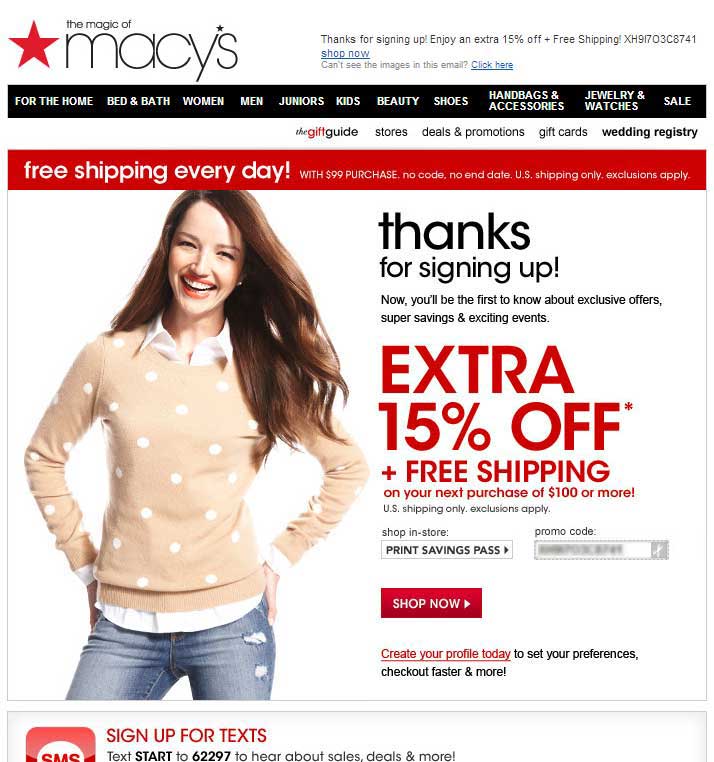This image depicts the homepage of Macy's, predominantly styled in black, white, and red hues, featuring a red Macy's star. The central theme of the page is "The Magic of Macy's." A welcoming message reads: "Thanks for signing up and enjoy an extra 15% off plus free shipping."

Navigation links are displayed for easy access to various categories: Home, Bed & Bath, Women, Men, Juniors, Kids, Beauty, Shoes, Handbags & Accessories, Jewelry & Watches, Sale, Gift Guide, Stores, Deals & Promotions, Gift Cards, Wedding Registry, and Free Shipping Every Day with a $99 Purchase (US Shipping Only; Exclusions Apply).

The main image showcases a woman with long red hair, wearing blue jeans, a white button-down shirt, and a light peach-colored sweater with white polka dots. She has a pale complexion and is pictured smiling.

A promotional text underneath the image states: "Thanks for signing up! Now you'll be the first to know about exclusive offers, super savings, and exciting events. Enjoy an extra 15% off plus free shipping on your next purchase of $100 or more (US shipping only; exclusions apply). Shop in store."

Below the text, there are buttons labeled "Print Savings Pass" and "Shop Now." Additionally, a promo code input field is blurred out. A red button labeled "Shop Now" is prominently displayed along with a prompt to "Create your profile today to set your preferences, check out faster, and more."